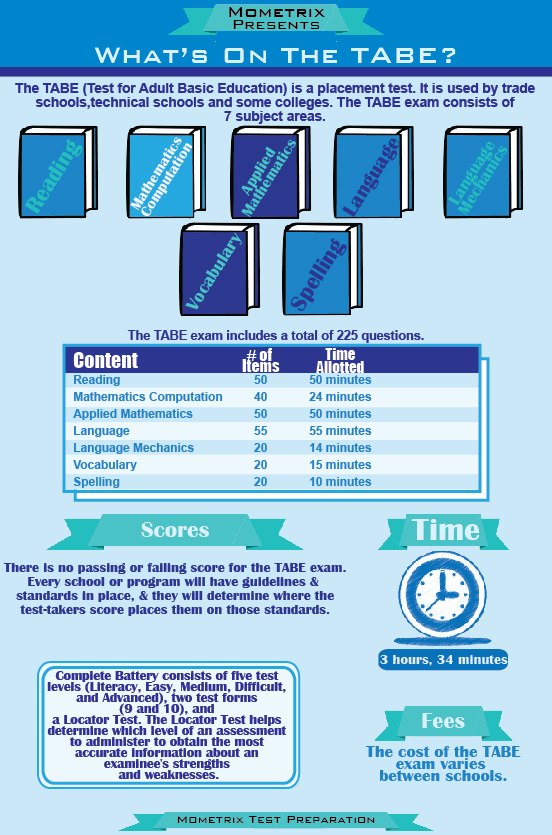The image is a detailed illustration primarily in shades of blue, resembling a poster. At the top, there's a dark blue rectangle that reads "MOMETRIX PRESENTS" in all capital, dark letters. Beneath it is a light green ribbon containing the text "WHAT'S ON THE TABLE?" in all capital white letters, followed by a light blue background.

The poster details the TABE (Test for Adult Basic Education) exam, a placement test used by trade schools, technical schools, and some colleges. The text explains that the TABE exam comprises seven subject areas, each represented by cartoonish blue books with visible white pages. Each book's title appears in varying fonts and colors:

1. **Reading** (dark blue book with light green font)
2. **Mathematics Computation** (lighter blue book with white font)
3. **Applied Mathematics** (dark blue book with light blue font)
4. **Language** (basic blue book with dark blue font)
5. **Language Mechanics** (same blue book with green font)
6. **Vocabulary** (dark blue book with light blue font)
7. **Spelling** (same blue book with dark blue font)

Below the books is a detailed table listing the subject areas, the number of items in each, and the time allotted for each section. The table headers are in a dark blue rectangle:

- **Content**: Reading, Mathematics Computation, Applied Mathematics, Language, Language Mechanics, Vocabulary, Spelling
- **Number of Items**: 50, 40, 50, 55, 20, 20, 20
- **Time Allotted**: 50 minutes, 24 minutes, 50 minutes, 55 minutes, 14 minutes, 15 minutes, 10 minutes

Each row in the table alternates between light blue and white backgrounds.

To the bottom left of the table, a light green ribbon says "SCORES" in white writing. The text explains that there is no passing or failing score for the TABE exam; guidelines and standards vary by institution to determine the placement of test takers.

To the lower right, another light green ribbon labeled "TIME" includes an image of a clock. The analog clock has a white outer rim, a blue middle, and a white center, showing the time at three o'clock and forty seconds. Below the clock is a rounded rectangle displaying "3 hours 34 minutes."

In the lower left, another white rectangle explains that the Complete Battery of the TABE consists of five test levels: Literacy, Easy, Medium, Difficult, and Advanced. It also details two test forms, 9 and 10, and describes the Locator test, which helps determine the appropriate test level to assess the strengths and weaknesses of the examinee accurately.

At the bottom, a ribbon notes that the cost of the TABE exam varies between schools. The entire illustration rests on a combination of white and light blue backgrounds, and at the very bottom, a banner reads "MOMETRIX TEST PREPARATION" in black writing.